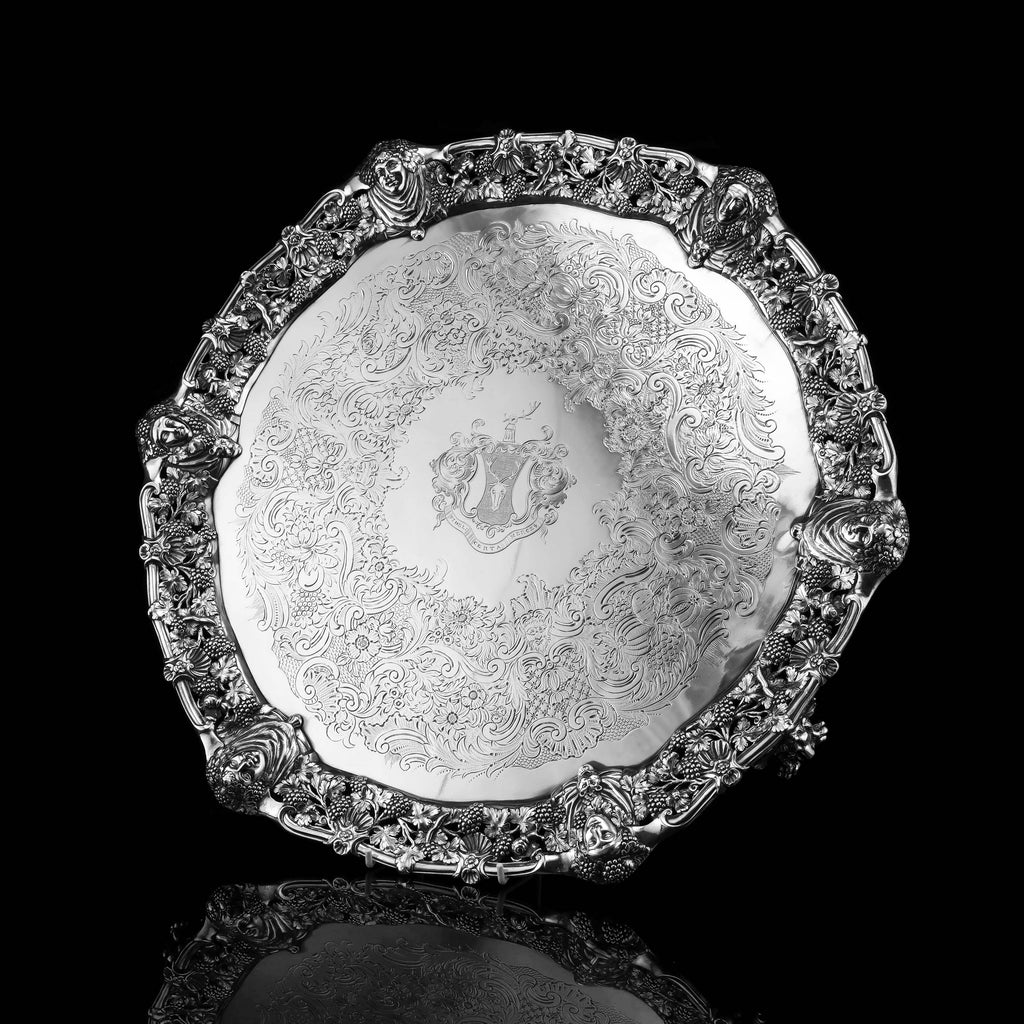This black-and-white photograph, taken indoors with artificial lighting, features a meticulously detailed and likely expensive silver disc showcased against a glossy black background, resulting in a distinct reflection at the bottom. The square image, which appears to have been carefully staged, depicts a large, circular object that might be a serving tray or possibly a decorative piece like the top of an ornate ring. The perimeter of the disc boasts a heavy-duty border adorned with intricate carvings, including faces, grapevines, and floral arrangements draped with scalloped linen. The lighter center of the tray displays a crest, surrounded by plain areas and further embellished with scalloped designs that resemble waves and leaves. Overall, both the craftsmanship and the rich detailing of the piece emphasize its possible high value and artistic significance.